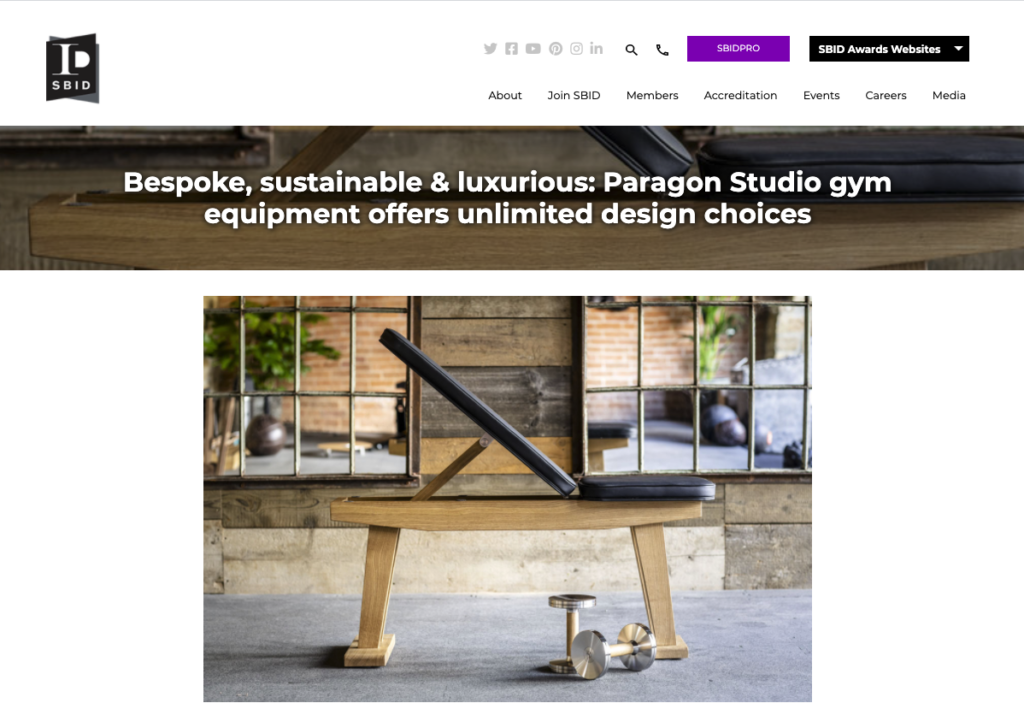Screenshot of the SBID website showcasing Bespoke Sustainable and Luxurious Paragon Studio Gym Equipment. The description reads, "Bespoke Sustainable and Luxurious Paragon Studio Gym Equipment Offers Unlimited Design Choices." Below the text is an image of a weight bench. The bench features a wooden frame with a padded, inclined seating area, highlighting an elegant design that combines form and function. The screenshot also includes a navigation bar at the top with clickable submenus labeled About, Join SBID Members, Accreditation, Events, Careers, and Media. Additionally, icons for social media platforms Twitter, Facebook, Pinterest, and Instagram allow users to connect with the brand. This company emphasizes the innovation of sustainable gym equipment, a concept not widely recognized before.